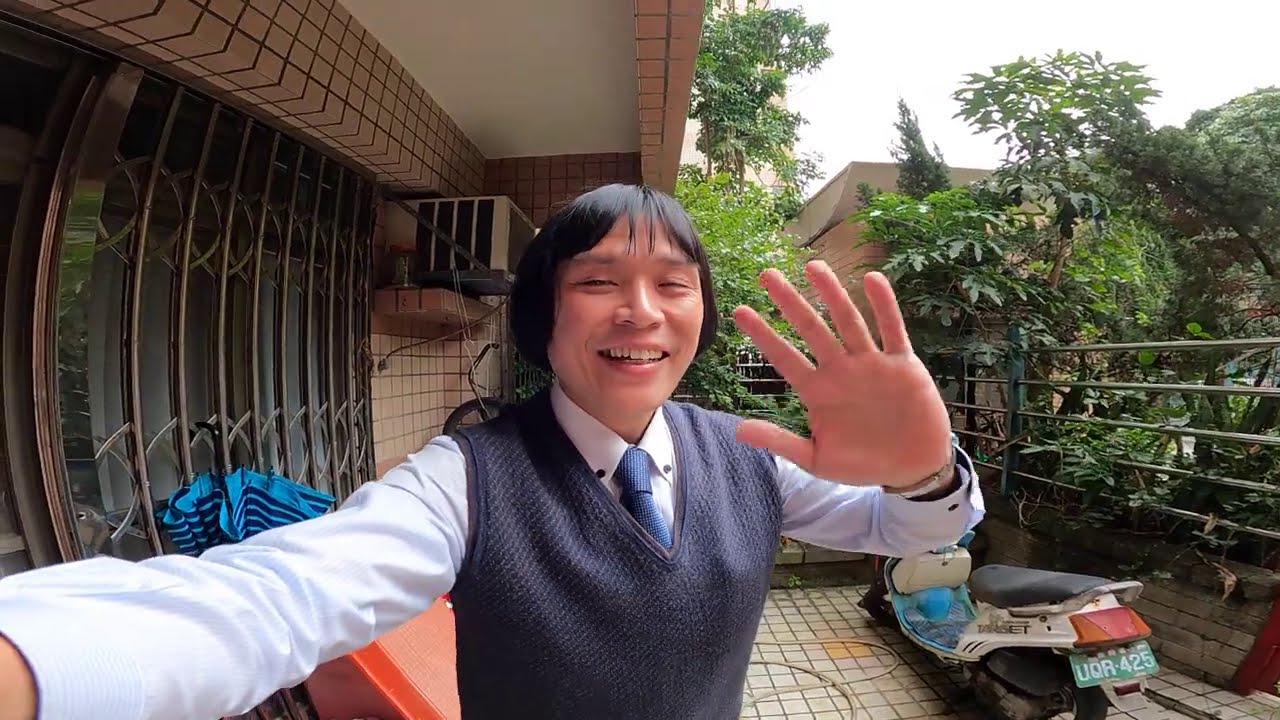In the center of this horizontal rectangular photograph, an Asian man with medium-length black hair and bangs is standing on the second-floor patio of a building. He is holding one hand up as if to say, “don’t take this picture,” while smiling and squinting his eyes, suggesting he knows the photographer. He is dressed in a white collared shirt, a blue tie secured with a tie pin, and a gray v-neck sweater. His other hand is partially extended, disappearing off-frame.

The patio features a white tile floor and white walls, with windows featuring metal bars along the left side. An air conditioning unit is visible in one of the windows. To the right of the man, the patio is bordered by a railing with trees and green foliage beyond it. A white and green moped with a black seat and a visible license plate sits just below the man’s left elbow, near some orange fencing. In the distance, through the trees, the rooftop of another house peeks out, contributing to the tropical atmosphere suggested by the abundant greenery.